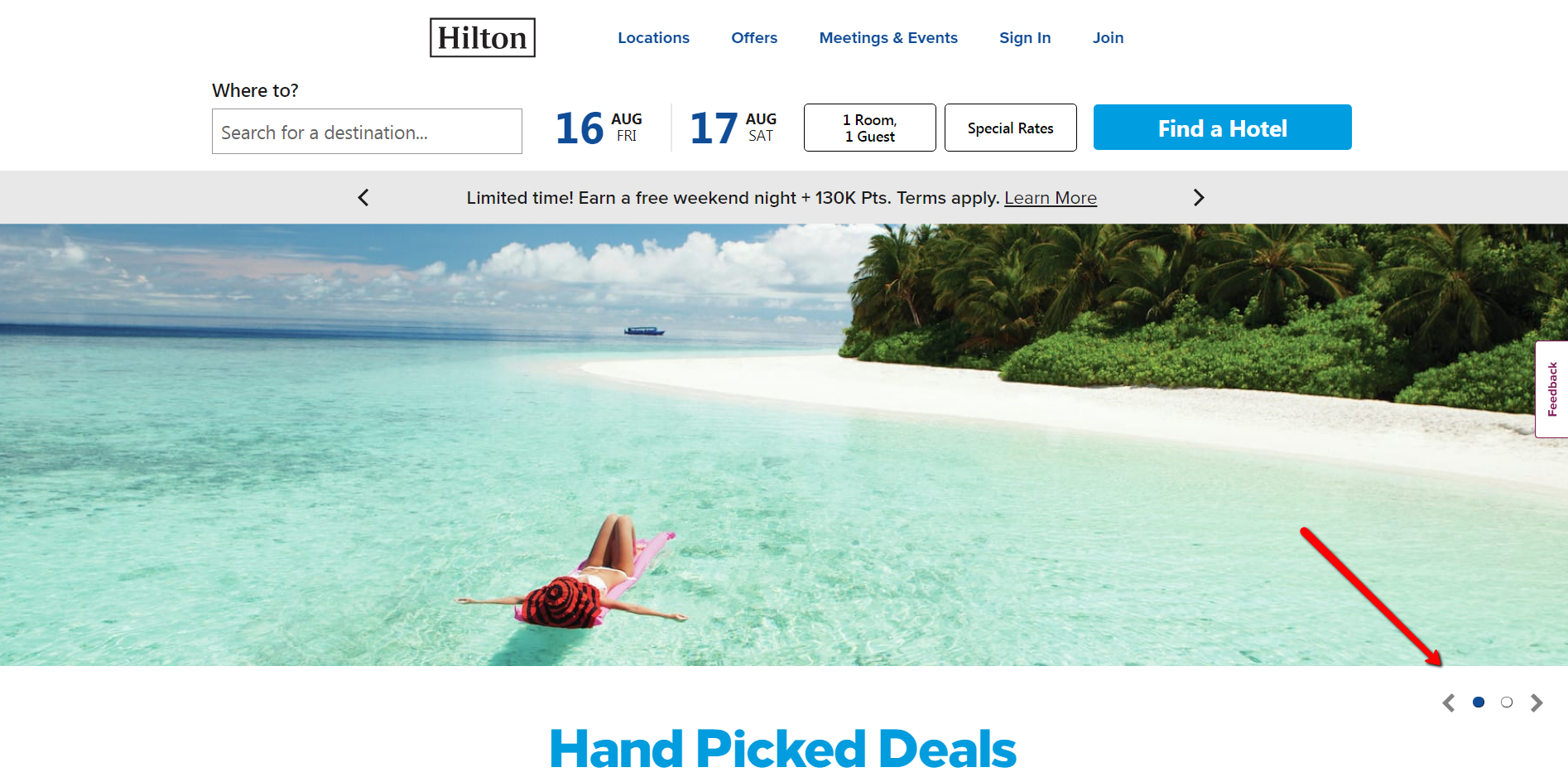The image showcases a serene beach scene with a woman leisurely floating on a pool float in the crystal-clear waters of a picturesque ocean. The water closest to the shore is a vibrant mix of light green and light blue, gradually transitioning into a deep blue hue towards the horizon. The background is dominated by a lush, tropical jungle that adds a touch of adventure and seclusion to the setting. The sky is mostly clear, with a patch of yellow and white clouds occupying about the top 20% of the image, though the clouds give way to the dense forest on the right side.

Overlaying this picturesque scene are various elements of a website interface. At the bottom of the screen, a banner reads “Hand-picked deals.” The top of the screen features “Hilton” along with navigational options such as Locations, Offers, Meetings & Events, Sign In, and Join. Just below this navigation bar, a search section invites users to explore destinations with a prompt "Where to?" accompanied by a calendar displaying dates: August 16th, Friday, and August 17th, Saturday. Additional search options include selecting the number of rooms and guests – defaulting to one room and one guest – as well as special rates, all contained within their respective rectangular boxes. A prominent blue button labeled “Find a Hotel” facilitates the search process.

Further down, before reaching the main image, a gray banner promotes a limited-time offer: "Earn a free weekend night plus 130,000 points. Terms apply. Learn more," enticing potential travelers with an attractive rewards package.